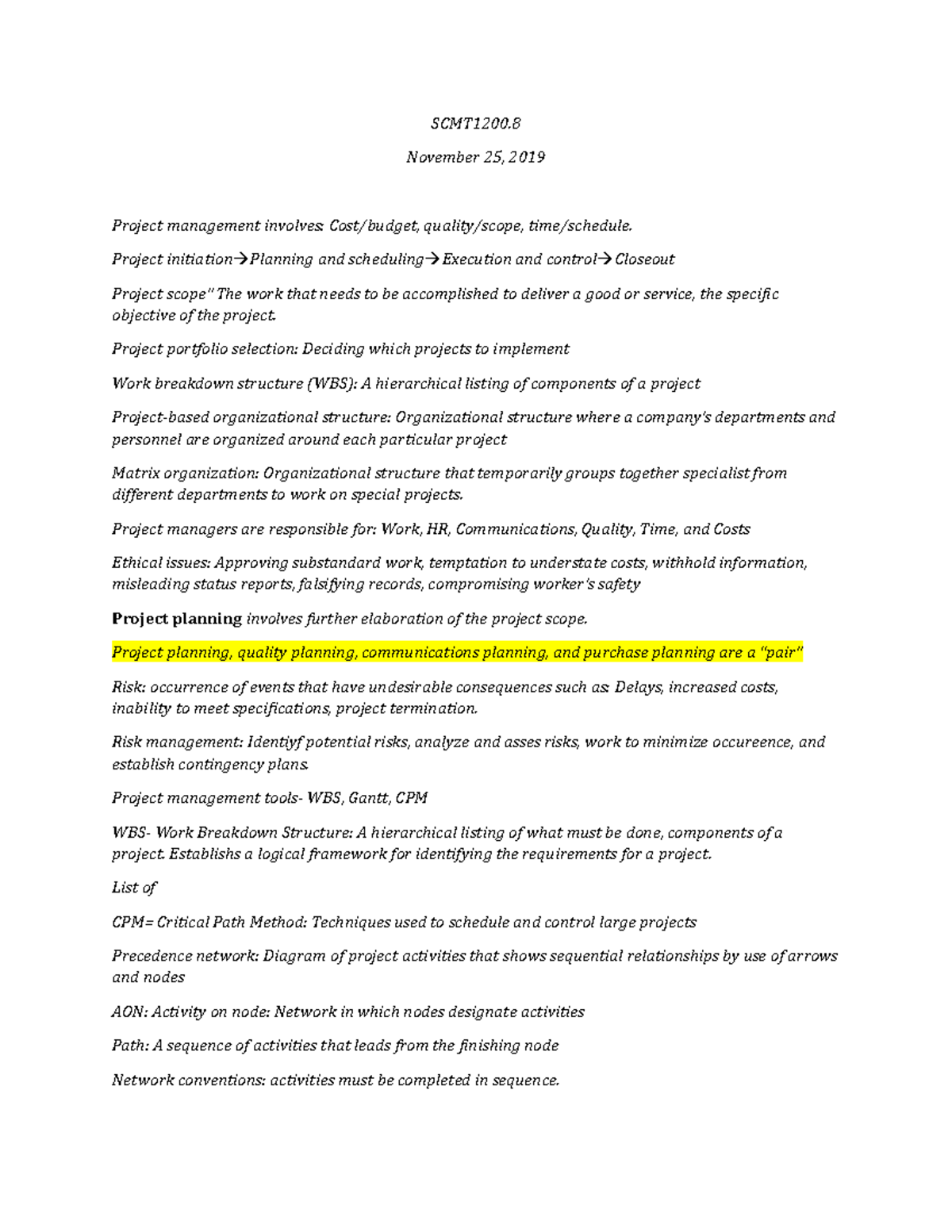Detailed Caption:

This image displays a comprehensive document on project management principles and methodologies, dated November 25, 2019, and identified at the top in bold capital letters as "SCMT 1200.8." The document is meticulously organized, featuring numerous lines of text outlining key concepts essential for effective project management. 

Highlighted in yellow, amidst the detailed text, is a specific line emphasizing the importance of project planning: "Project planning, quality planning, communications planning, and purchase planning are a 'pair.'"

The document begins with a foundational definition: "Project management involves: cost/budget, quality/scope, time/schedule." It then meticulously breaks down the phases of project management, starting from initiation leading to planning and scheduling, progressing to execution and control, and concluding with closeout.

Highlighted topics include:
- **Project Scope:** Defines the work required, including the delivery of goods or services, and outlines specific objectives.
- **Project Portfolio Selection:** Methods for deciding which projects to implement.
- **Work Breakdown Structure (WBS):** A hierarchical listing of a project's components.
- **Project-Based Organizational Structure:** Describes how companies organize departments and personnel around specific projects.
- **Matrix Organization:** Details how specialists from various departments collaborate on special project tasks.
- **Responsibilities of Project Managers:** Highlights duties across work, human resources, communications, quality, time, and costs.

Additionally, the document addresses ethical issues in project management such as approving substandard work, the temptation to underestimate costs, withholding information, misleading status reports, falsifying records, and compromising worker safety.

Key phrases are bolded for emphasis, such as "Project planning involves further elaboration of the project scope," and various project management tools and techniques are listed, including the Critical Path Method (CPM), precedence networks, activity-on-node (AON) representations, path, and network conventions.

Overall, the document serves as an in-depth guide covering the essential elements and methodologies critical to successful project management.